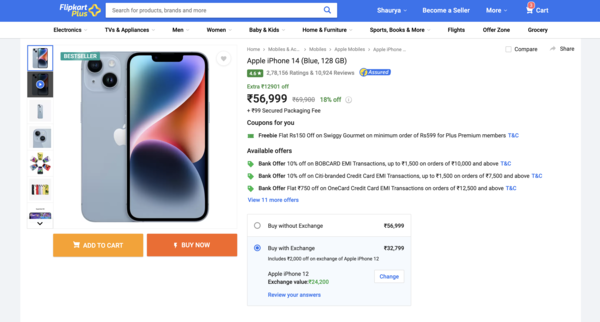We are viewing an e-commerce website with a heavy focus on detailed navigation and product presentation. At the top, there's a partially obscured logo possibly reading "something plus," alongside a search bar and a navigation bar with various categories such as Electronics, TV and Appliances, Men, Women, Boy or Baby and Kids, Home and Furniture, Sports, Books, and more.

Centered prominently is a display section featuring the Apple iPhone 14, showcasing both front and back views of the device. Additional images of the iPhone are available for those seeking more visual details. Below the images, there are two prominent orange buttons: "Add to Cart" and "Buy Now," suggesting immediate purchasing options for convenience-driven customers.

This section also highlights an enticing offer for another Apple product, the iPhone 12 with 128GB of storage, priced at £56,999. The colorful layout features a blue-themed header and orange accents at the bottom, contributing to a vibrant and engaging user experience. This site appears to prioritize both aesthetic appeal and functionality, aimed at providing an optimized shopping experience.